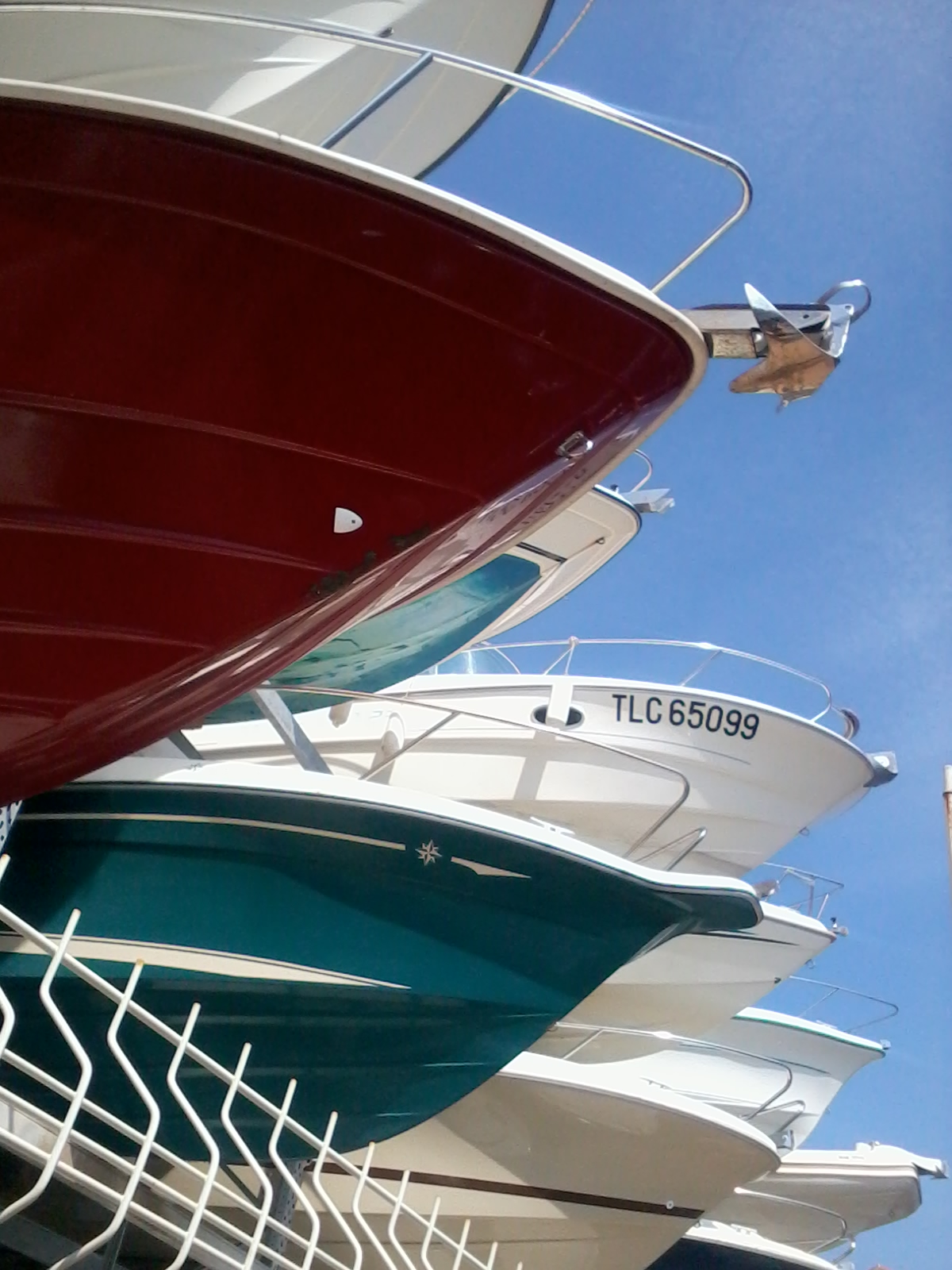The image captures a striking upward view of a tiered storage facility filled with various boats against a clear, blue sky. In the foreground, occupying the upper left, is a boat with a dark amber, maroon-colored hull, accentuated by a white trim and a silver piece protruding from its center. This boat features a distinctive white speck in the middle and a metal handrail at the front. Adjacent to it is a light teal boat, decorated with white lines and a star emblem near the top, also equipped with a steel handrail. Further to the right, there is a white boat marked with black letters reading "TLC 65099," joining several other pure white boats lined up with visible metal handrails. At the bottom corners of the image, a white barrier with pointed barbs is noticeable, presumably to prevent unauthorized crossing. An anchor dangles from one of the boats, adding to the marine atmosphere of the scene.